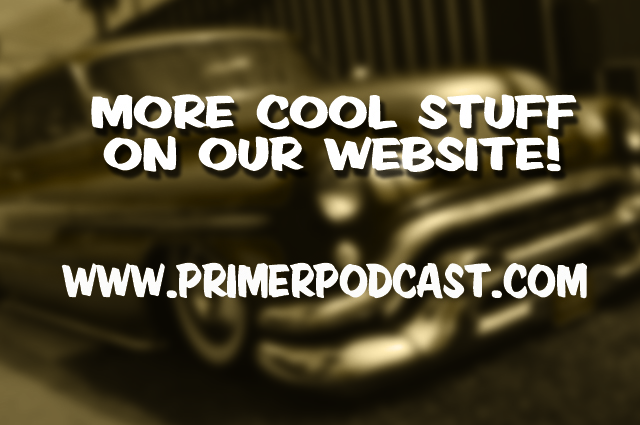The image presents a predominantly gold-brown background featuring a blurred photograph of an old-fashioned car, likely from the 1940s. This vintage vehicle, notable for its large bumper, whitewall tires, and topless design, sits against what might be a backdrop of fencing on the right side. Overlaid on this retro scene is a promotional text in white font with a black shadow effect that adds depth. The text reads, "More cool stuff on our website, www.primerpodcast.com" (spelled out as P-R-I-M-E-R-P-O-D-C-A-S-T). The design aims to draw attention to the classic car while directing viewers to visit the podcast website.